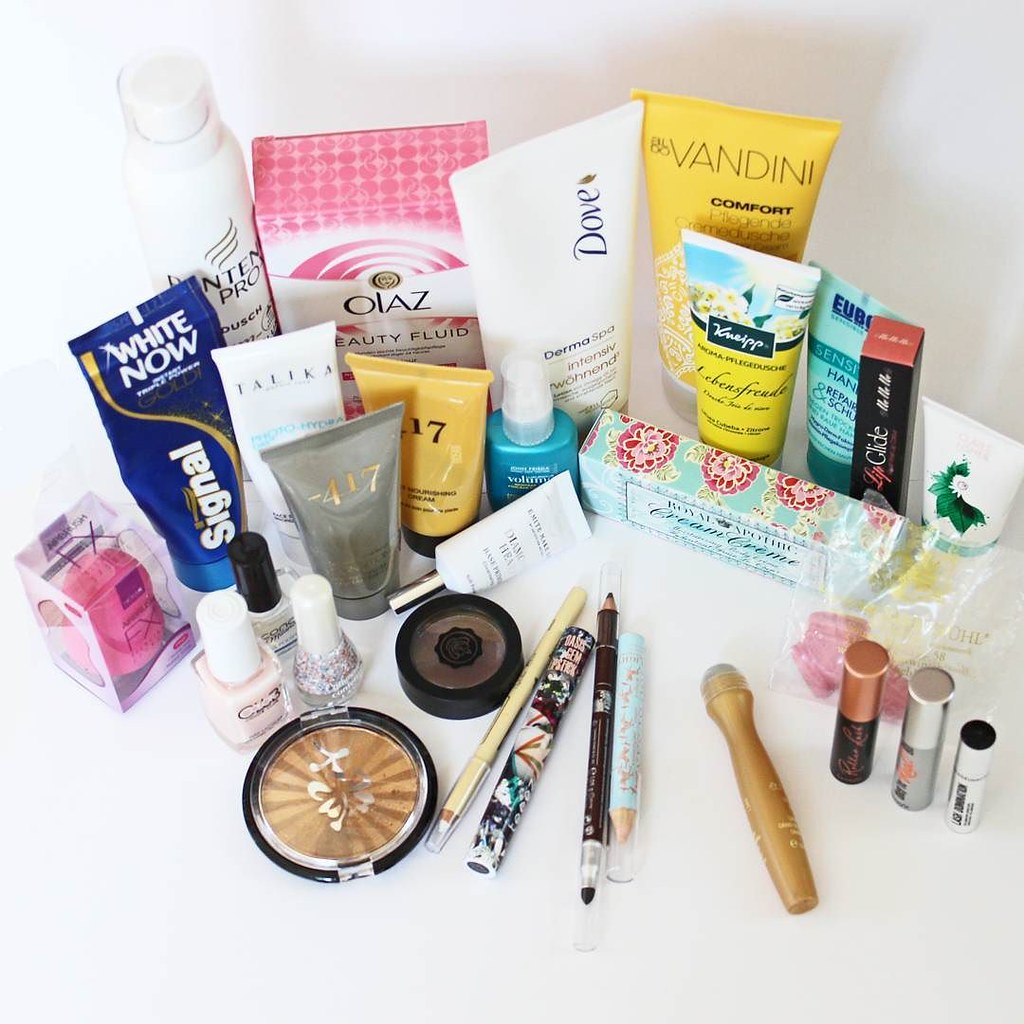The image displays a cluttered bathroom counter, featuring various makeup, skincare, and hair care items against a white backdrop. The viewpoint is from above, providing a comprehensive look at the assortment spread across the white counter. Starting from the left:

1. **Beauty Blender Sponge**: Still in its see-through box, marked with "FX," showcasing the pink sponge inside.
2. **Toothpaste**: Metallic blue tube labeled "Signal White Now," adorned with a gold swirl design, standing upright.
3. **Pantene Pro-V**: Resembling dry shampoo, in a white bottle positioned in the back row.
4. **Olay Beauty Fluid**: In a box with pink dots and swirls on a white background, prominently displayed.
5. **Dove DermaSpa Lotion**: Situated in the back, it indicates "Intensely" on the bottle, suggesting its lotion type.
6. **Vandini Comfort Lotion**: Bright yellow, matching the height of the Dove bottle, also in the back row.
7. **Flowers-Adorned Lotion**: Smaller lotion bottle, featuring floral designs on top and a yellow label below.
8. **Teal Travel Lotion**: Compact and travel-sized.
9. **Lipstick Box**: Black base with a taupe pink top, indicating the shade of the lipstick inside.
10. **Tiny Travel Lotion**: Another small lotion bottle positioned on the far-right side.

In the middle row:

11. **Pink Earplugs**: Possibly within a bag, indicated by the pink contents inside.
12. **Fancy Cream in a Box**: Box adorned with pink peonies on an aqua background.
13. **Travel Items**: Blue, yellow, gray, and white containers, mostly standing, accompanied by a small white tube.
14. **Nail Polishes**: Three neutral-colored polishes in front of the toothpaste, one with a glittery finish; two with white brush handles, one with a black handle.
15. **Bronzer**: Circular bronzer resembling a circus tent design, with alternating shades and a silver symbol.
16. **Brown Eye Shadow**: Compact in a black container, adjacent to the bronzer.

In the front row:

17. **White Eyeliner**: Simple liner likely used for defining the eyes.
18. **Abstract Lipstick**: Another lipstick, this one in a uniquely designed container.
19. **Lip Liner Pen**: Used for defining the lips.
20. **Aqua Concealer Pencil**: Possibly for spot treating.
21. **Golden Rollerball Applicator**: An applicator, likely for serums or oils.
22. **Travel-Size Mascaras**: Three Benefit brand mascaras, the first in black and rose gold, the second and third in silver.

The array of items reflects a well-used and varied collection of personal care products, all meticulously arranged within the limited space of a bathroom counter.